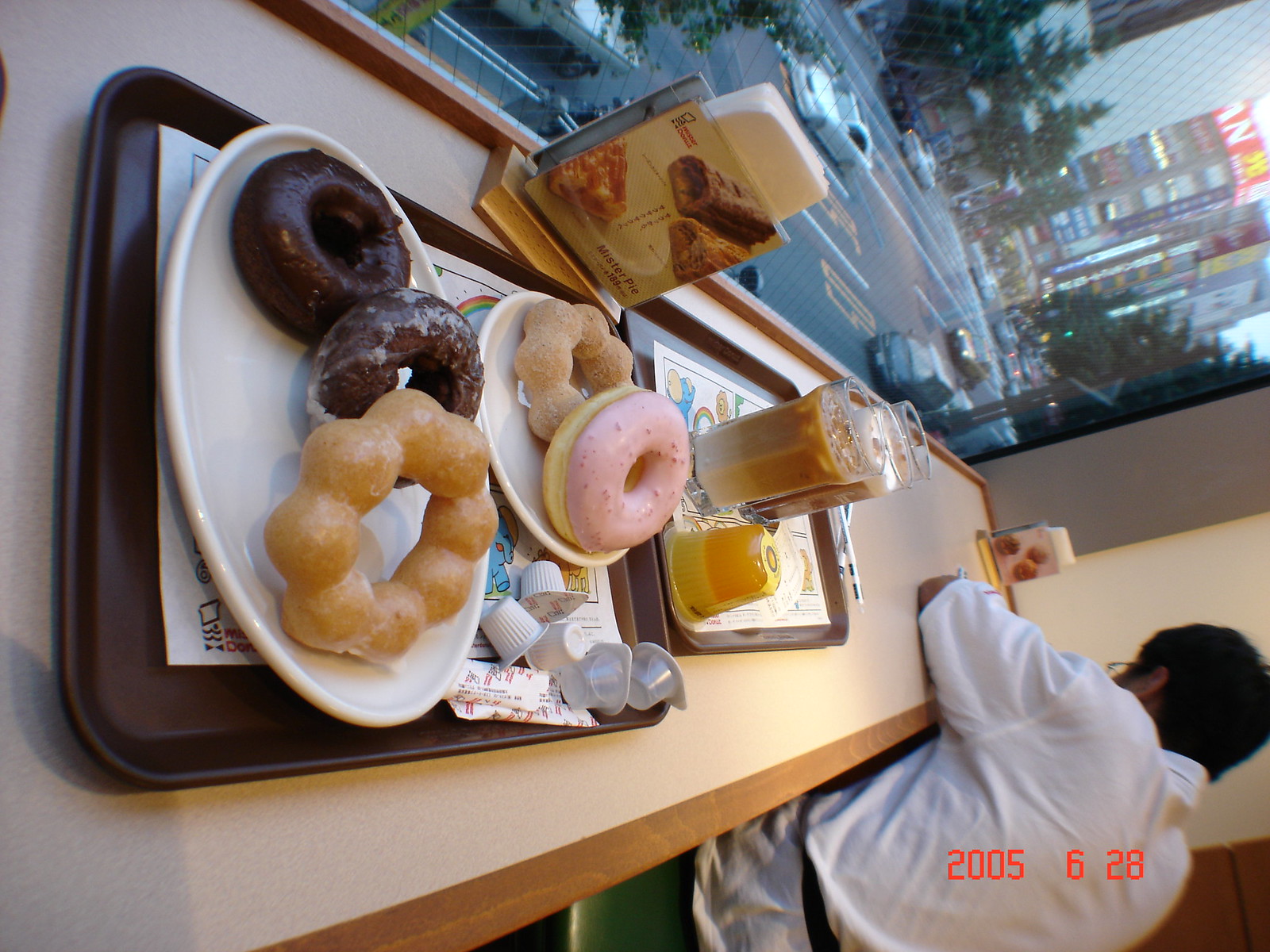The photograph, taken and time-stamped on 2005-06-28, appears to be a somewhat aged Polaroid-style image of a Mr. Donut shop, likely at the Akihabara location in Japan, suggested by the visible Japanese lettering and the busy urban scene with skyscrapers, trees, and cars outside the window. Despite being sideways in orientation, the image captures a detailed breakfast counter scene. There are two trays: the left tray holds two white plates with donuts - the larger plate boasting three donuts, two chocolate-glazed and one larger plain mochi donut composed of small balls forming a ring. The smaller plate on the same tray contains a smaller version of the plain mochi donut and a pink frosted cake donut. The right tray features three iced coffees or glass cups filled with drinks, along with a flan or pudding and numerous coffee creamers. A man with glasses can be seen on the far right, partially visible as he looks down, possibly seated at the counter decorated with table flags displaying images of pastries and donuts, one of which is labeled "Mr. Pie." The counter itself is white with a light tan rim, reflecting the café's simple yet cozy ambiance.